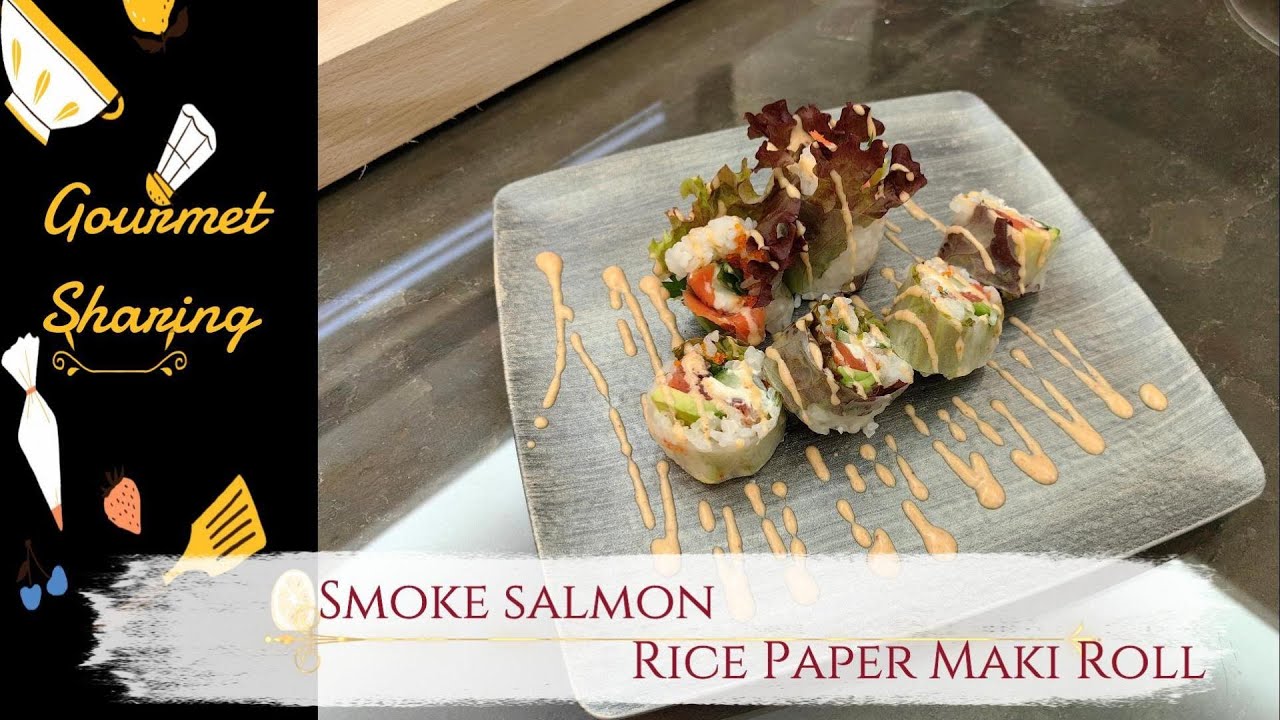The image portrays a gourmet presentation of smoked salmon rice paper maki rolls. Displayed on a sleek, gray square plate with slightly rounded edges, the tray holds six pieces of the maki roll, meticulously arranged. The rolls feature an appetizing mix of white rice, vibrant orange smoked salmon, fresh green vegetables, and brown seaweed, creating a colorful and inviting dish.

Aesthetically plated, the maki rolls are garnished with a large lettuce leaf and artistically drizzled with an orange sauce, adding a decorative and flavorful element. The plate rests on a dark brown marble table, enhancing the dish's elegant presentation.

On the left side of the image, a strip labeled "Gourmet Sharing" in yellow lettering includes simple illustrations of various kitchen tools—a spatula, an icing pipette bag, a salt shaker, a bowl, a cup, a strawberry, and some blueberries—highlighting the culinary theme. The text "Smoked Salmon Rice Paper" is prominently displayed at the bottom in red, emphasizing the dish's key ingredients and gourmet appeal.